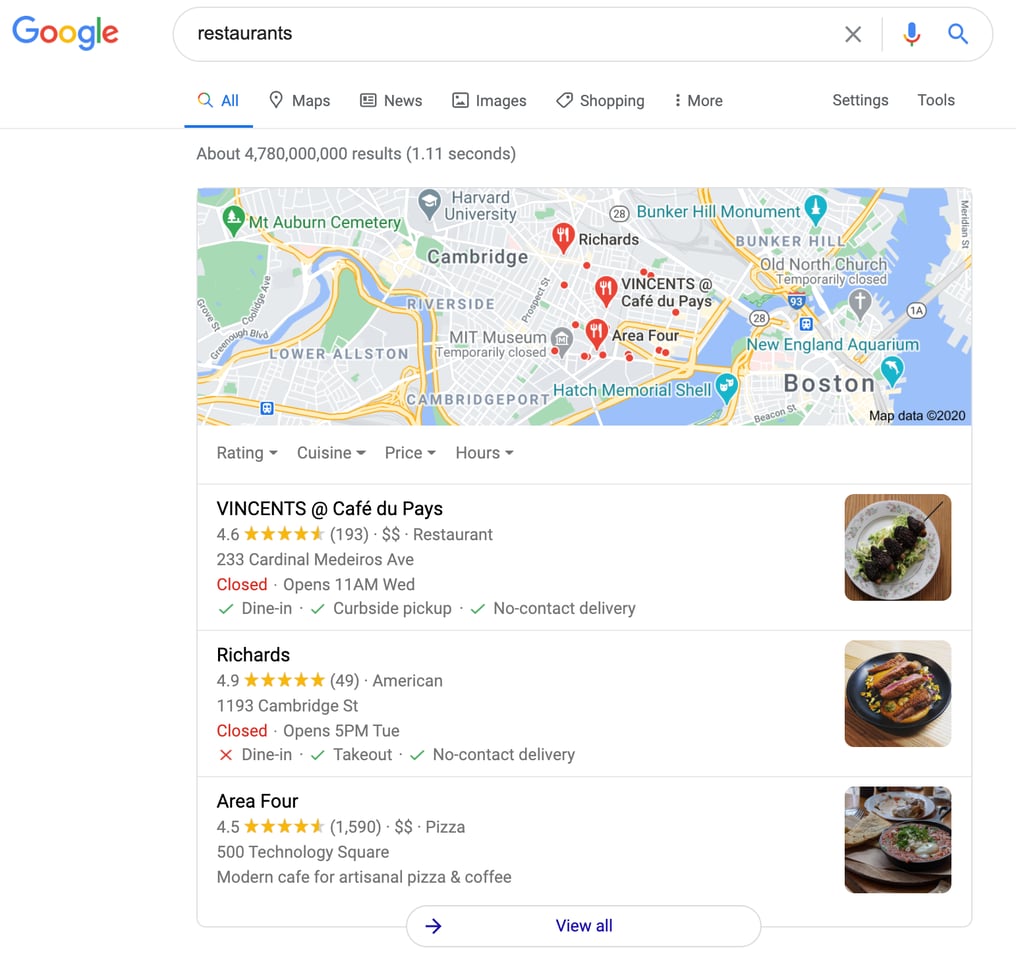The image showcases a Google search result for "restaurants," featuring the Google logo in the upper left corner and the familiar search bar at the top. The results seem to focus on the Boston and Cambridge area, with a map highlighting notable locations such as Cambridge, Harvard University, Boston, New England Aquarium, Bunker Hill, and Bunker Hill Monument.

A list of restaurants is displayed, including detailed information about each establishment. Vincent's at Cafe DuPage, located at 233 Cardinal Madreas Avenue, has a rating of 4.6 stars. The image indicates that it is currently closed and will reopen at 11 a.m. on Wednesday. Richard's, situated at 1193 Cambridge Street, offers American cuisine and boasts an impressive 4.9 out of 5 stars.

Another restaurant listed is Area 4, found at 500 Technology Square, known for its modern café setting and artisanal pizza and coffee offerings. Each restaurant listing is accompanied by a thumbnail image of a dish, providing a visual preview of the cuisine.